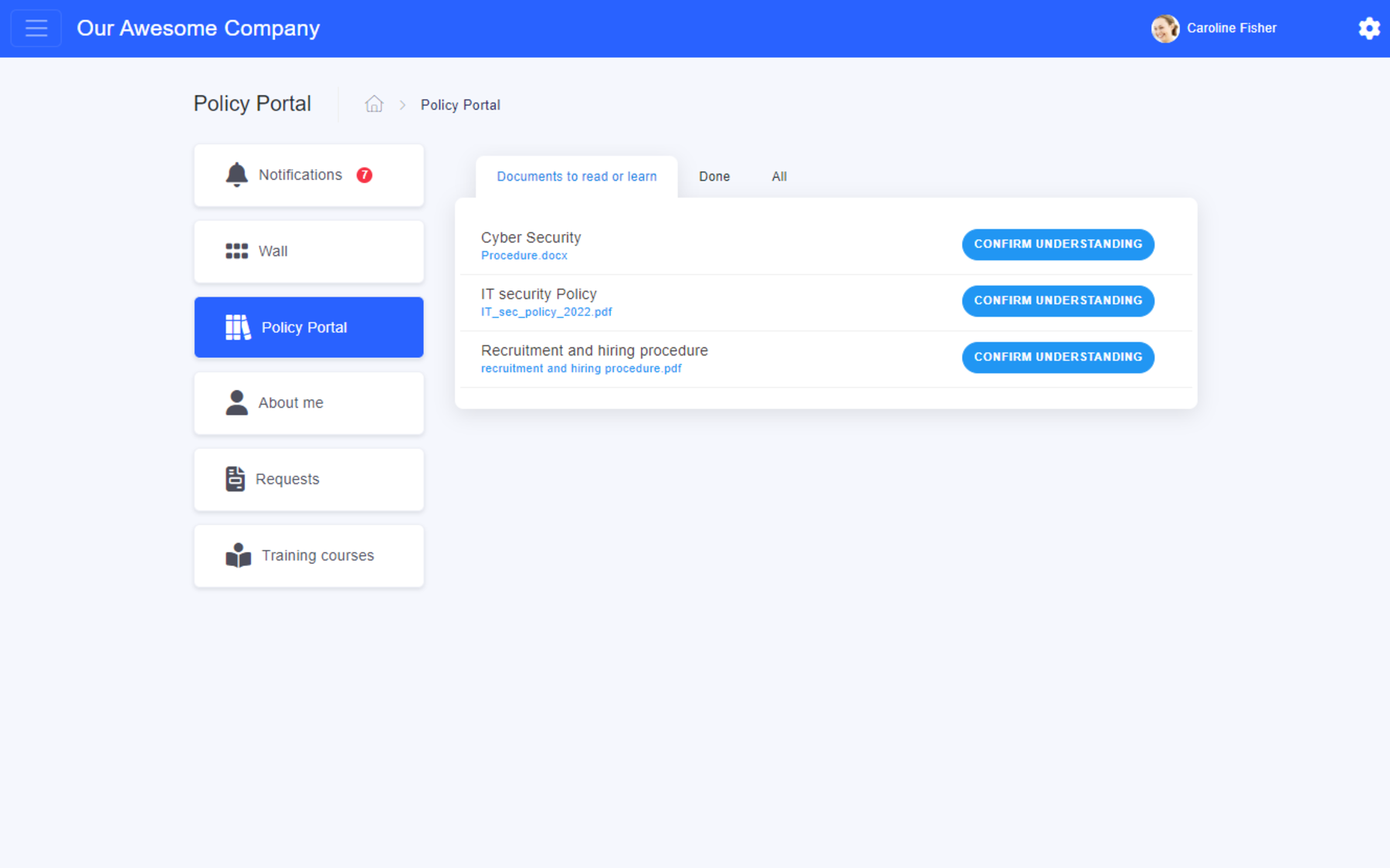This image showcases a digital dashboard interface from 'Our Awesome Company.' In the top left corner, a menu bar is visible, featuring several key sections: Policy Portal, Notifications (indicating seven unread notifications), Accounts, Requests, Training Courses, Documents to Read or Learn, Cyber Security, and several confirmed understandings of critical company policies such as IT Security Policy and Recruitment and Hiring Procedure. The layout is clean and organized, highlighting the company's commitment to structured information access and employee engagement in policy adherence and professional development.